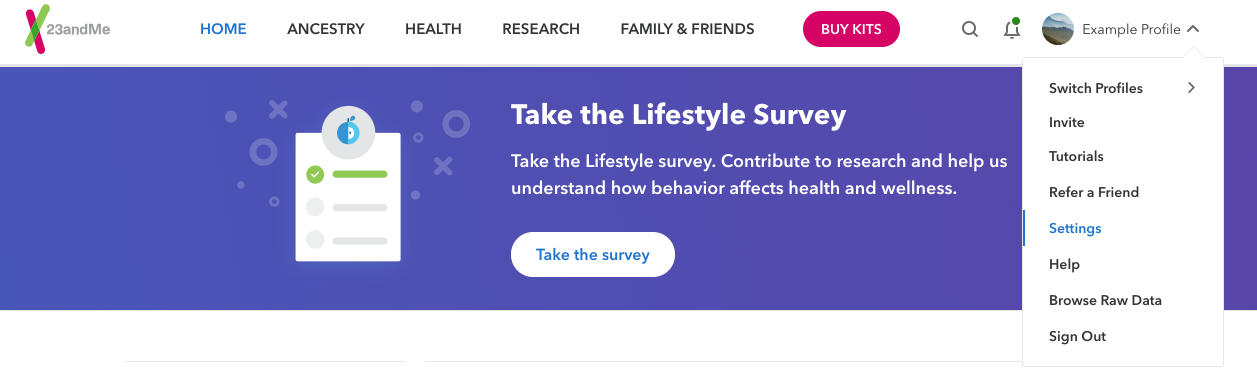Screenshot of the 23andMe user interface against a white background. A prominent pink and green 'X' logo is positioned centrally. The interface displays multiple tabs: 'Home,' 'Ancestry,' 'Health,' 'Research,' 'Family & Friends,' each accessible from the top navigation bar. A red oval button labeled 'Buy Kits' stands out vividly in white text. 

To the right, there is a magnifying glass icon for search functionality next to a notification icon with a green dot, denoting new activity. Adjacent to these icons is a round profile picture placeholder labeled 'Example Profile.'

Beneath this, a purple rectangle section features a white checklist icon, indicating tasks or surveys. One item highlighted in green urges users to 'Take the Lifestyle Survey,' which encourages participation in research to enhance understanding of behavior’s impact on health and wellness. A white oval button beneath this invites users with blue text, 'Take the Survey.'

On the left sidebar, beneath a white box titled 'Switch Profiles,' there are quick access options in blue text: 'Invite,' 'Tutorials,' 'Refer a Friend,' 'Settings,' 'Help,' 'Browse Raw Data,' and 'Sign Out,' providing easy navigation for account management and additional features.